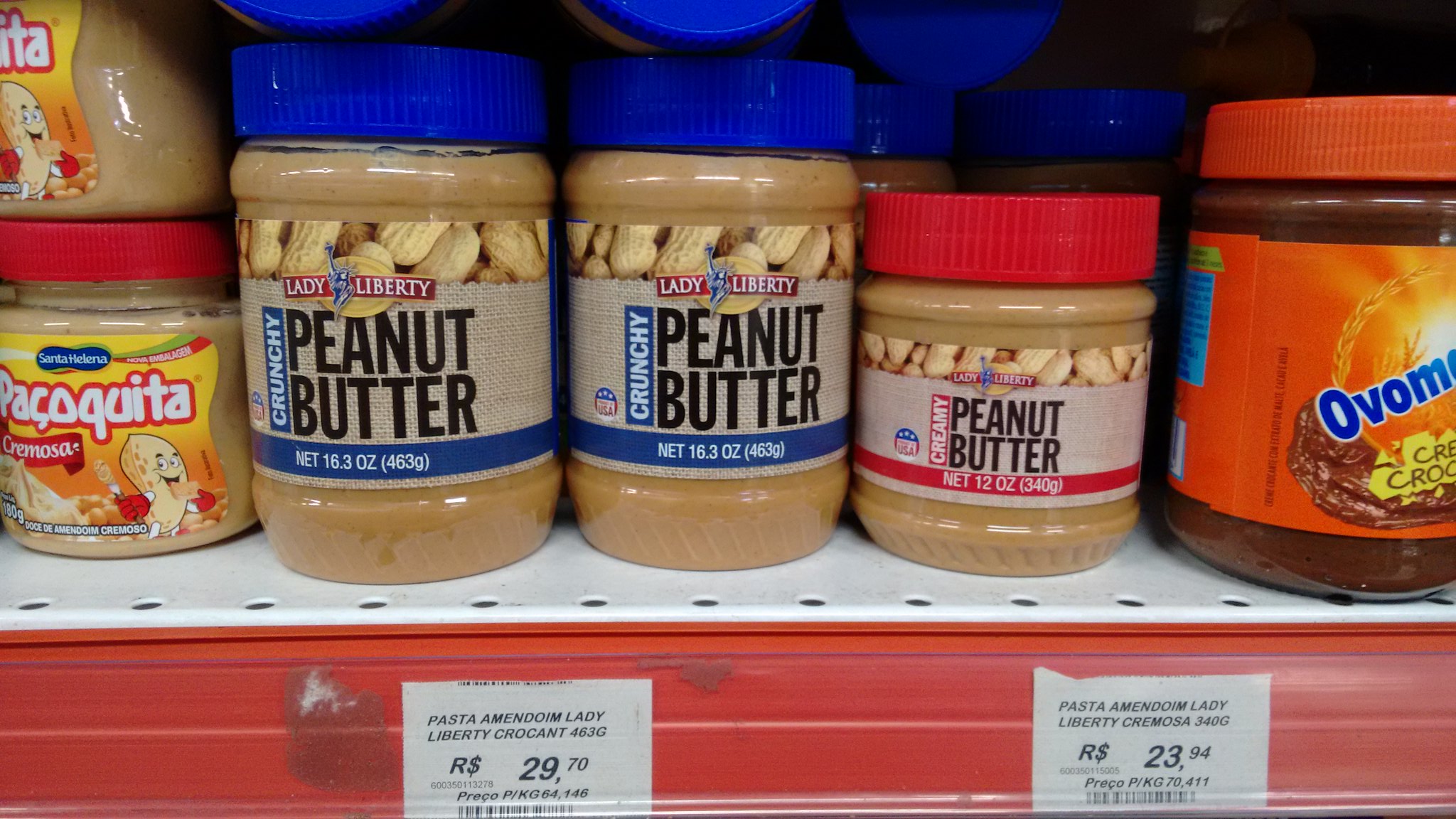The photograph is a wide-angled image taken in a supermarket, focusing on a shelf stocked with various brands of peanut butter. The lower portion of the image includes a red plastic shelving unit with visible price tags. On the left side of the bottom shelf, there is Pasta Lady Liberty Croquant priced at $29.70. On the right side, there is Pasta Amedeum Lady Liberty Cremosa, 340 grams, priced at $23.94. 

The majority of the image showcases six jars of peanut butter arranged on the shelf. On the far left, there are two jars of Paquita peanut butter. Centrally on the left side, there is a jar of Peanut Butter Crunchy Lady Liberty. To its immediate right is a jar of Peanut Butter Creamy Lady Liberty. Lastly, on the far right, there is a jar of Ovamo, which appears to be a creamy chocolate-flavored spread.